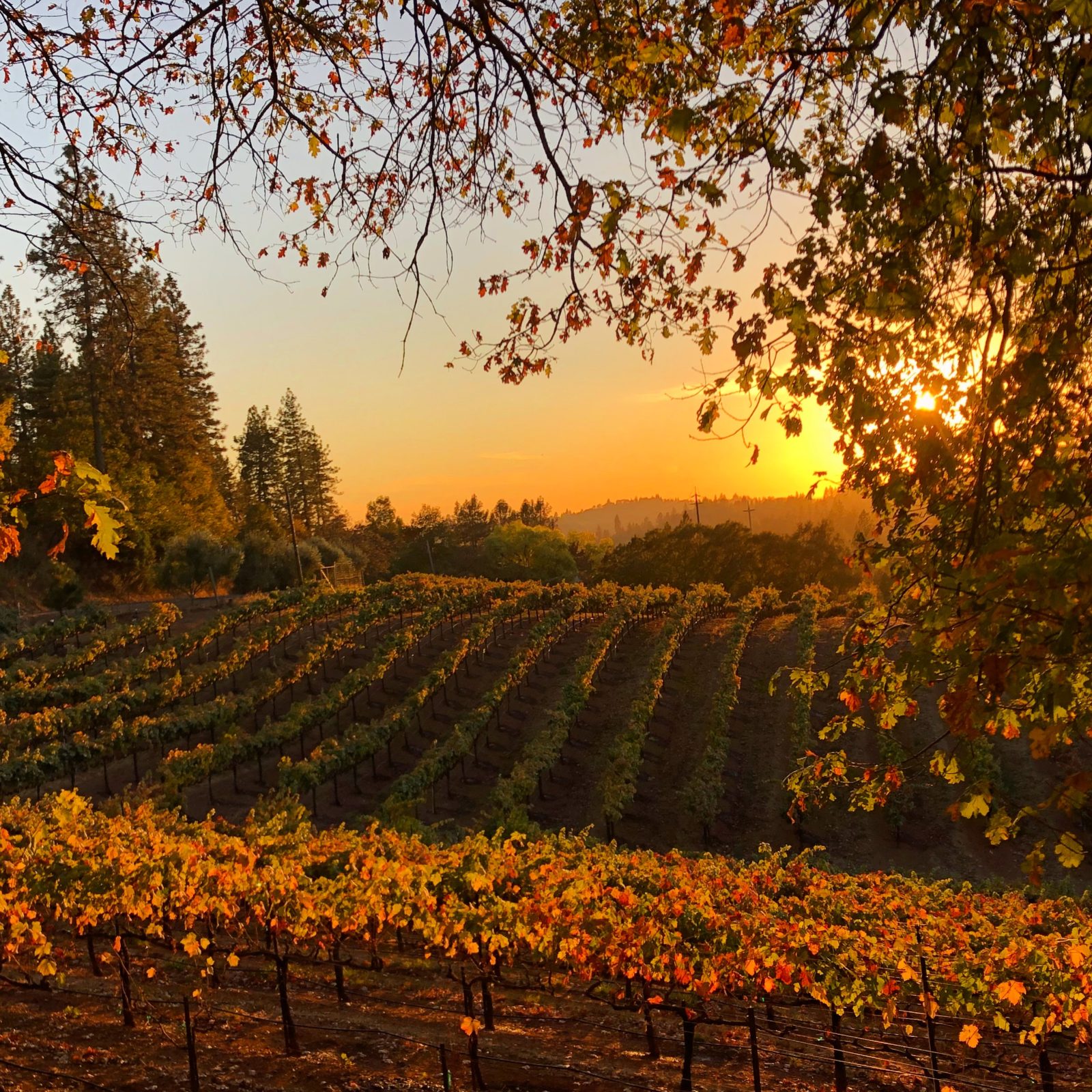This photograph captures a picturesque vineyard at sunset, characterized by rows of small trees or vines, suggesting some sort of fruit crop, possibly grapes, planted in straight, vertical lines. The field is on a sloped hill that descends and then rises back up, creating a varied terrain. The rich, green plants contrast vividly with the brown soil that fills the spaces between the rows, and there are at least 14 distinct rows visible. Surrounding the vineyard, on both the left and right sides, are dense forests of pine trees and large green bushes, framing the agricultural scene. In the background, the landscape includes a mix of trees and open soil patches extending towards a distant hill that spans horizontally across the horizon. The sky is an orangey-yellow gradient melting into a very light blue or almost gray above, and the setting sun behind some trees on the right side appears intensely bright, casting a golden hue over the entire scene.